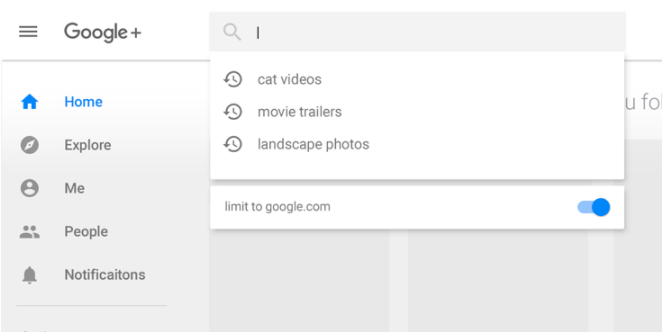This panoramic image depicts a screenshot of a website, capturing a section of a Google+ interface. On the upper left, there are three elongated gray bars, beneath which lies the Google logo displayed in gray, accompanied by a gray plus symbol to its right. Adjacent to this, a truncated gray bar extends further to the right but gets cut off by an overlay, suggesting an active selection or click.

At the very top of the image, a gray bar extends across, containing a magnifying glass icon on the right side, representing the search functionality. Within this search bar, the capital letter "I" is present. Directly below, a white section features a clock icon labeled "cat videos" in gray. This is followed by another clock icon with "movie trailers" and then yet another with "landscape photos," all in gray.

A narrow gray bar divides these sections from a white bar beneath it, displaying a gray text that reads "limit to google.com." To the right of this, a prominent blue toggle switch is visible.

Towards the left side of the image, a blue house icon labeled "home" signifies the active selection. Underneath this icon, there is a gray circle with a white diamond-like shape and the text "explore." Adjacent to this is another gray circle containing a person icon labeled "me," followed by an icon representing two people labeled "people." The next icon is a bell symbol labeled "notifications." Below this sequence, three additional gray bars remain blank, adding to the minimalist design.

In the top-right corner, partially obscured by another box mentioned earlier, are the letters "you fo" in gray, indicating text that extends beyond the visible area.

Overall, this image captures various elements of a navigation menu within the Google+ interface, providing a detailed view of its layout and components.